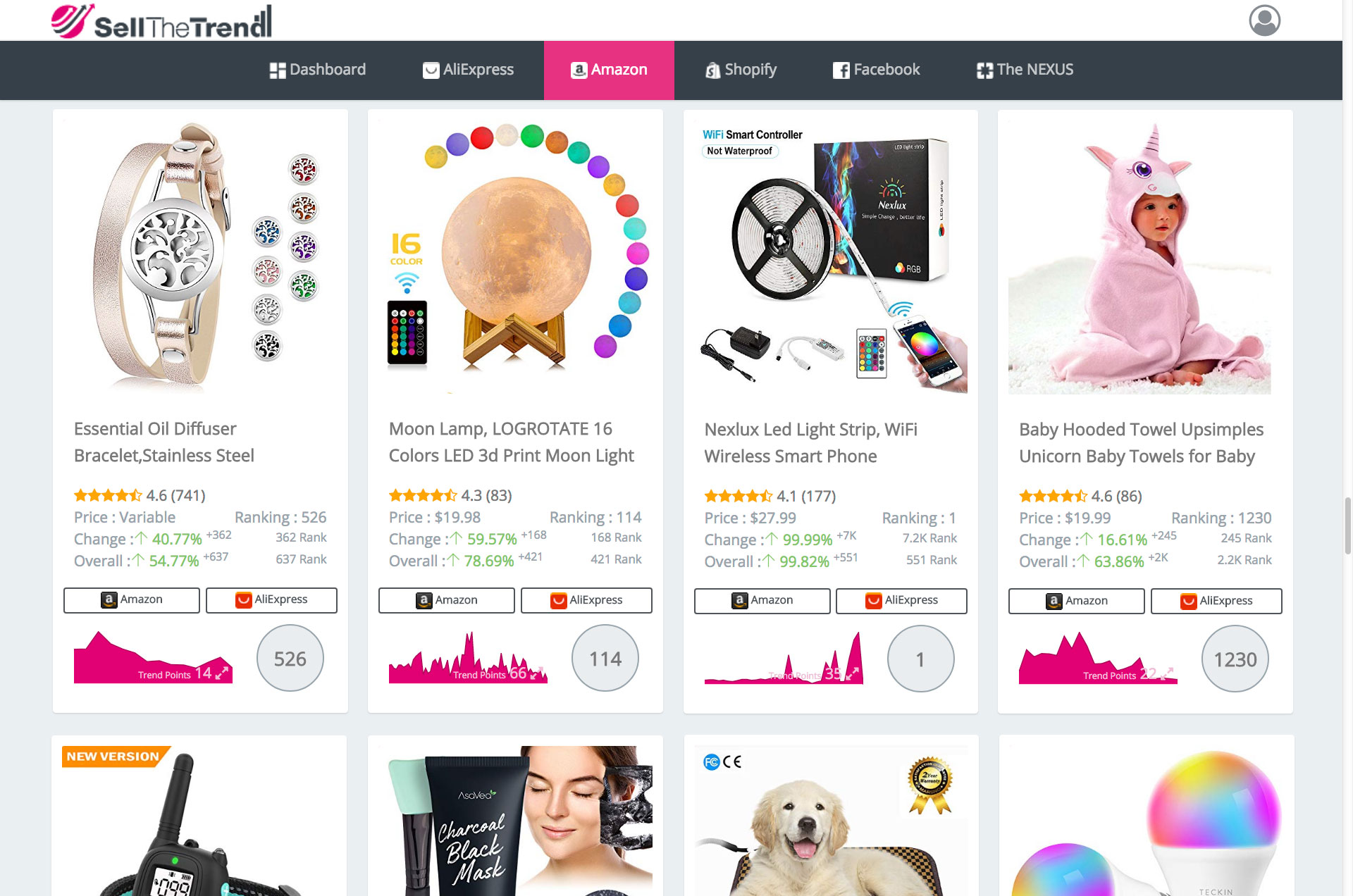On the shopping page, the upper left corner features a stylish pink and black logo with the text "Sell The Trend" displayed prominently beside it. In the upper right corner, there is a profile login icon for user account access. Below this, the page is divided into two rows of four product images each, though the second row is partially cut off from view.

The top row showcases four distinct products, each accompanied by descriptive text, numerical ratings, and a chart for reference. 

1. The first image presents a product that resembles a watch but is identified in the description as a "Stainless Steel Essential Oil Diffuser Bracelet." This bracelet features customizable options with several small interchangeable circles in different colors displayed next to it. 

2. The second image depicts the "Logrotate 16-Colors LED 3D Print Moon Lamp." This innovative lamp is designed to look like a moon and is set on a wooden holder. Surrounding the lamp are several small circles displaying the various color options available for the LED light. 

These detailed and visually engaging product descriptions aim to attract potential buyers by clearly illustrating the unique features and customization options available for each item.